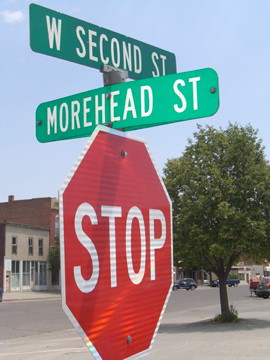This daytime photograph features exceptional image quality and presents a detailed urban scene. In the foreground, a prominent red and white stop sign is clearly visible, adorned with two green street signs with white lettering. The bottom sign reads "Moorhead Street," while the top sign indicates "West 2nd Street."

The background showcases a lush, green leafy tree with a sturdy brown trunk casting shadows beneath it. The city street behind is dotted with several cars, including a gray vehicle and a blue one, along with additional cars parked along the sides.

Further back, two buildings can be seen prominently on one side: a tan building with visible windows and an adjacent brick structure. Opposite, other buildings of varying tan shades are discernible. The sky is a clear blue, and part of a white structure is faintly visible, adding to the urban landscape’s depth and dimension.